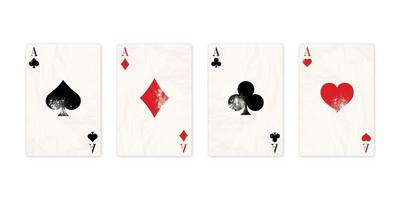The image depicts a set of four aging playing cards arranged in a horizontal row against a solid white background. Each card is an ace, featuring the ace of spades, ace of diamonds, ace of clubs, and ace of hearts, from left to right. The card faces are predominantly white, with slightly larger suit symbols prominently displayed in the center of each card, exhibiting noticeable wear and faded edges, indicative of sun damage or frequent use. In the upper left and turned upside down on the lower right corners of each card, the letter 'A' and its respective suit symbol are printed. The overall arrangement and wear give the cards an antique appearance.